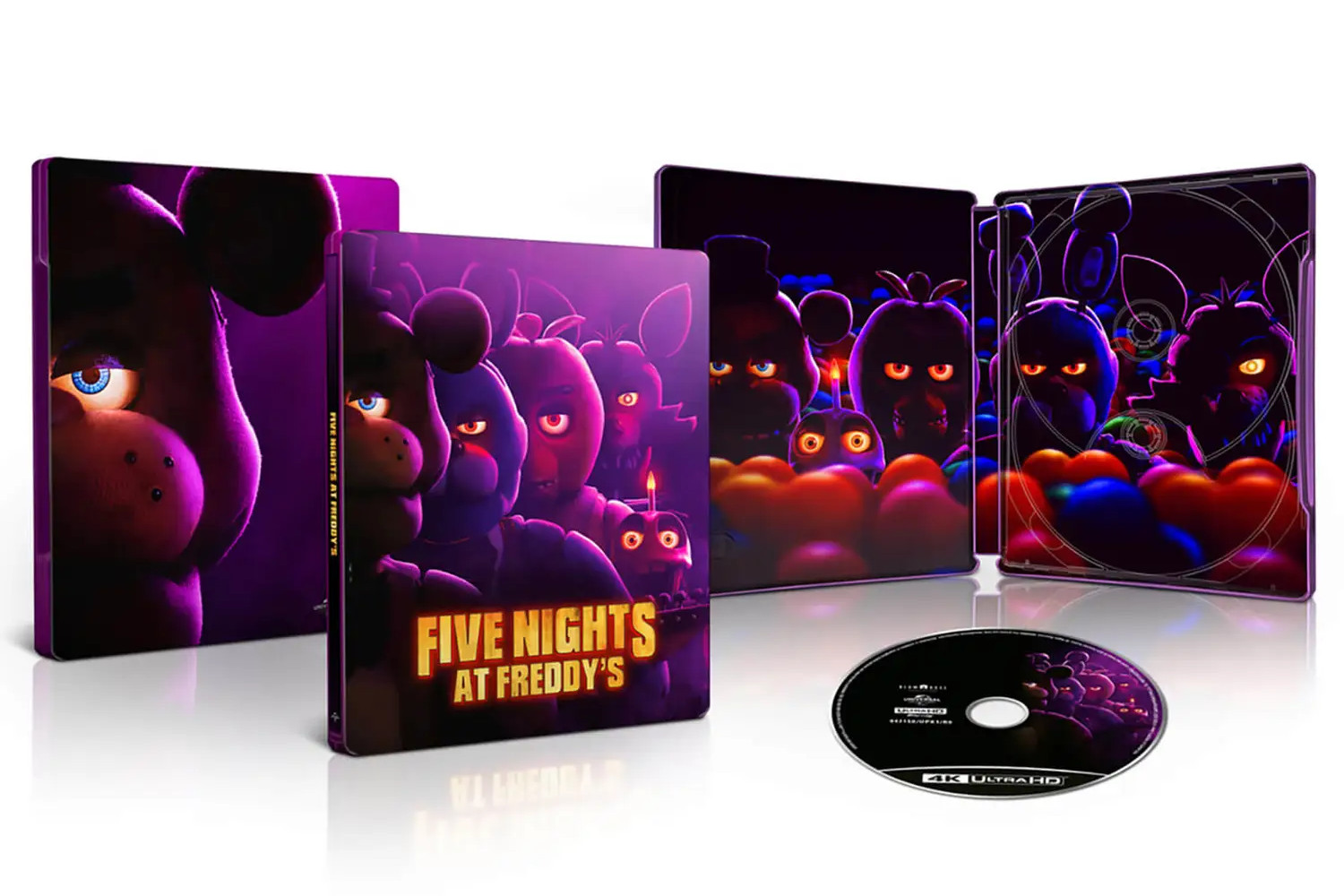Against a stark white background, this image showcases the DVD case for the horror film based on the video game Five Nights at Freddy's. The cover prominently features an eerie color scheme of purples, blues, deep reds, and blacks. Displayed on the cover are various unsettling animatronic characters, notably a blue bear, a mischievous rabbit, and another bear-like figure. One of these characters is particularly distinctive, sporting a candle with eyes and teeth on its head. The characters possess striking eyes, with hues varying from yellow to orange and blue. Accompanying the DVD case is a black disc labeled "4K Ultra HD," which bears the same haunting imagery as the cover. In the backdrop, a folded booklet mimics the cover design, underscored by the vibrant yet terrifying characters of the Five Nights at Freddy's universe. The overall arrangement and the various elements emphasize the horror and detailed artistry associated with this franchise.